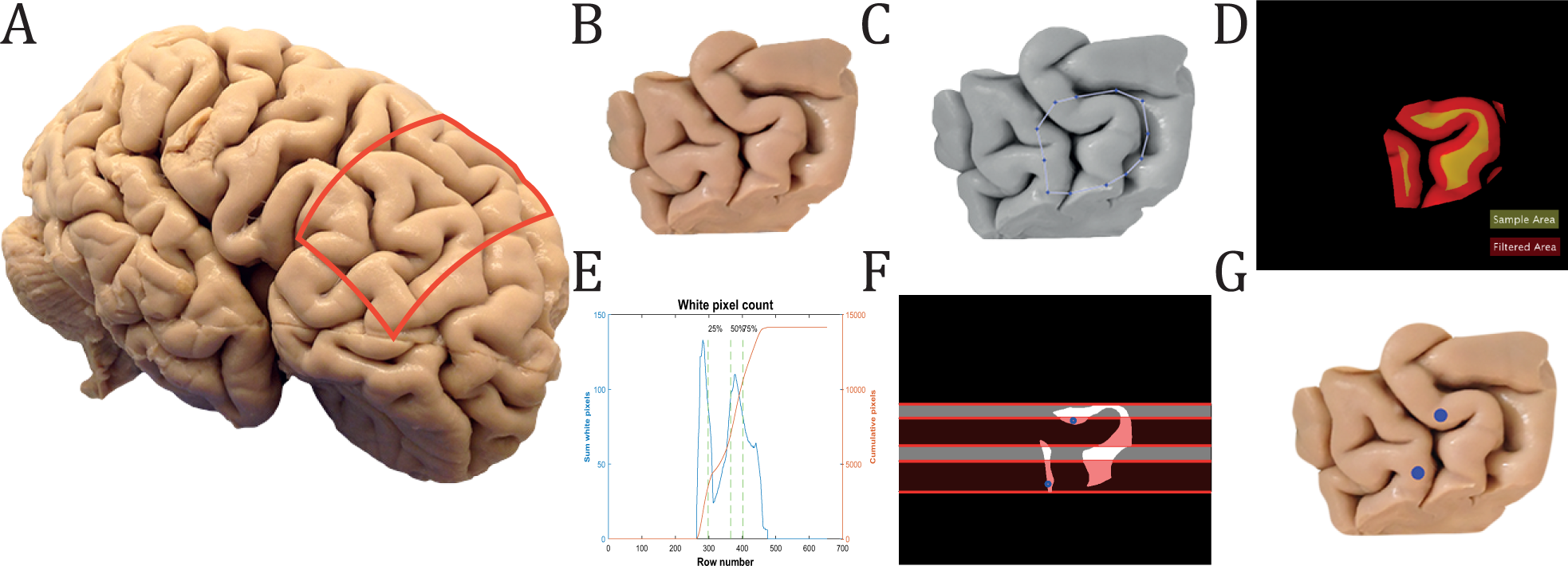The composite image series, labeled A through G, provides a detailed examination of a human brain through various imaging techniques. Image A, the largest on the left, depicts a typical nude-colored human brain with a noticeable red square highlighting a section in the upper back right area. Image B zooms in on this highlighted brain section, showing it in more detailed cross-section. Image C presents the same cross-section as B but in gray, with a small section circled in blue. Image D amplifies this small section, displaying it in red and yellow on a black background to emphasize specific features, almost resembling an imaging scan, accompanied by illegible text in the bottom right corner. Image E, directly below B, is a line graph titled "White Pixel Count," illustrating values with an X and Y axis, though specifics remain unclear. Image F reverts to the cross-section from C and D, this time in black, with white brain matter intersected by five horizontal, semi-transparent red laser-like lines. The final image, G, mirrors the gray cross-section of B but now marked with two blue dots in the center of the focus area.